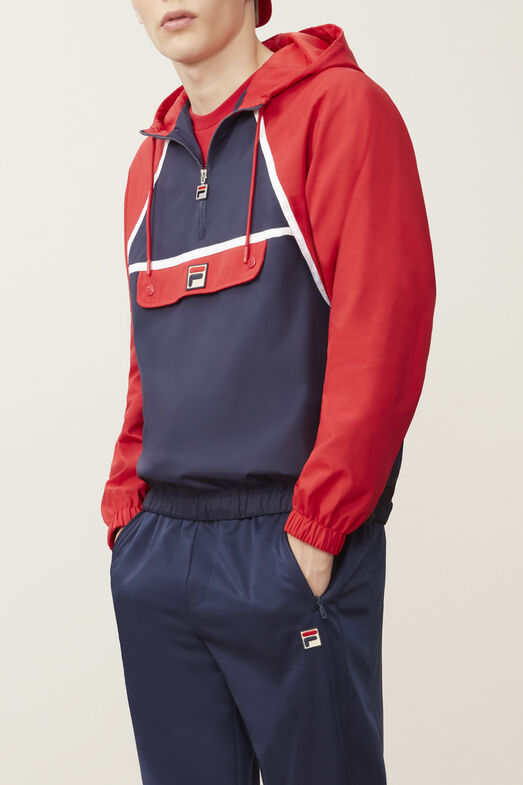This photograph features a close-up of a male model dressed in a stylish jogging outfit. From the visible details, we see him from just below his nose down to his thighs. His pose is casual with both hands placed in his pockets, and although his body is angled toward the left, he gazes straight ahead. The expression on his slightly parted lips reveals a hint of light pink. His ensemble consists of dark blue running pants and a coordinating sweatshirt, which sports red sleeves and a zipper that extends halfway down. The sweatshirt also includes pull strings adorned with a red element, alongside a prominent 'F' logo, where the top stripe is red and the bottom part is dark blue. The backdrop is a plain beige, keeping the focus solely on his figure. The image exudes a modern, athletic vibe, possibly representing a brand associated with the FIFA logo.